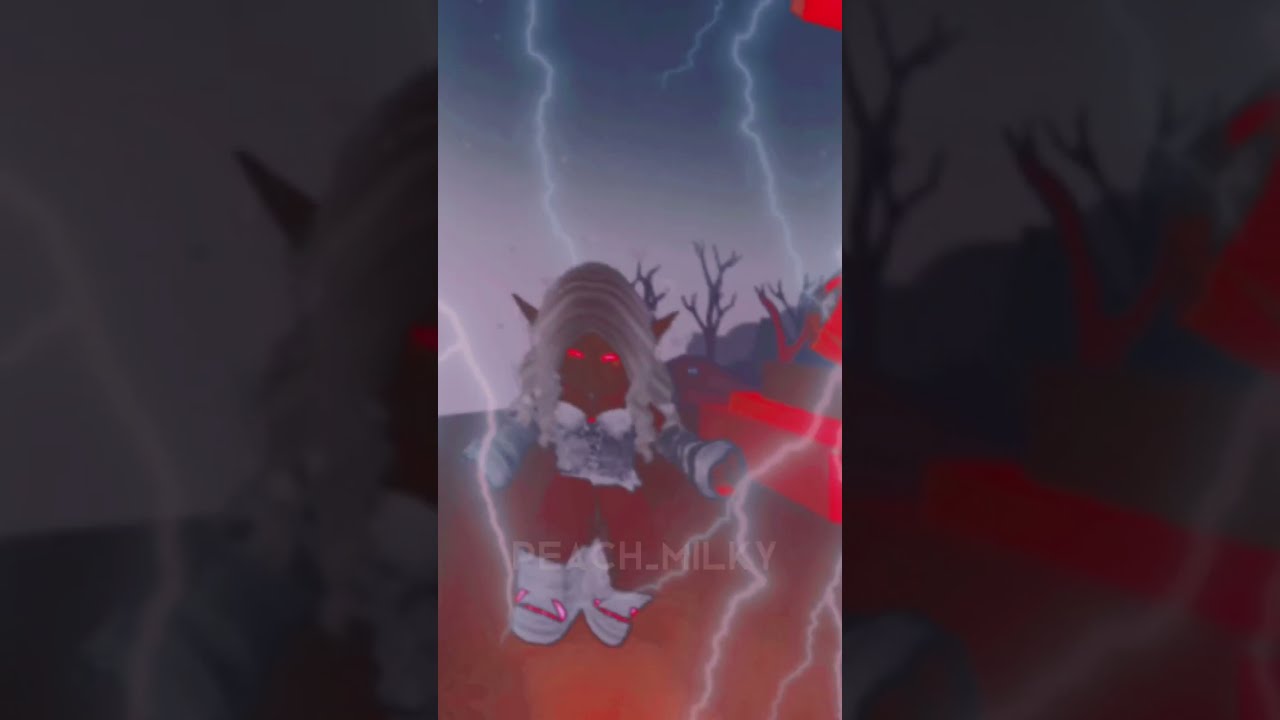The image appears to be a detailed illustration or a screenshot from a comic book, cartoon, or video game, depicting a striking and mysterious character. This animated figure, resembling a humanoid creature, is positioned on the left side of a landscape that combines elements of desert and spooky forest. The character has very dark skin contrasted sharply by long, white-gray hair, and glowing bright red eyes. Distinctive sharp elven-like ears stick out from each side of its head, adding to its otherworldly appearance.

The figure is dressed in a white and gray dressy shirt with a corset featuring a red diamond in the middle, red pants, and chunky white tennis shoes. It stands amidst a scene filled with eerie details such as leafless trees, red blocks, and possibly coffins, all under a stormy sky laced with striking lightning bolts.

The overall palette of the image is dark, with hues of blues, reds, blacks, and grays, contributing to its spooky, vampiric vibe. There is a watermark on the image, which reads "peach_milky" located in the center near the bottom. The vivid animation and intricate background details, including the semi-transparent lightning and various gloomy elements, make the image a captivating piece of artwork.